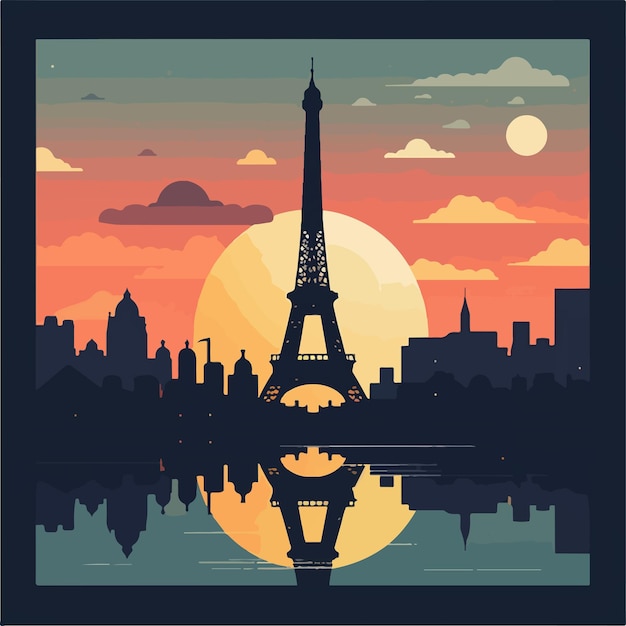This digital graphic is a mesmerizing illustration of Paris, France, featuring a silhouette of the iconic Eiffel Tower standing majestically against a vibrant sunset backdrop. The sky is a stunning blend of colors, ranging from maroon to peach, with clouds in hues of gray, yellow, and orange. Behind the Eiffel Tower, a large, glowing yellow-orange sun sets, casting a warm, radiant light across the scene. To the upper right, a circular bright object, possibly the moon, adds another layer of intrigue to the sky. Surrounding the Eiffel Tower are silhouettes of various buildings, emphasizing the city's distinctive skyline. Below, a body of water mirrors the entire picturesque scene—the Eiffel Tower, the sun, and the cityscape—creating a beautiful, symmetrical reflection. The overall composition of the image captures the timeless beauty and grandeur of Paris during sunset.